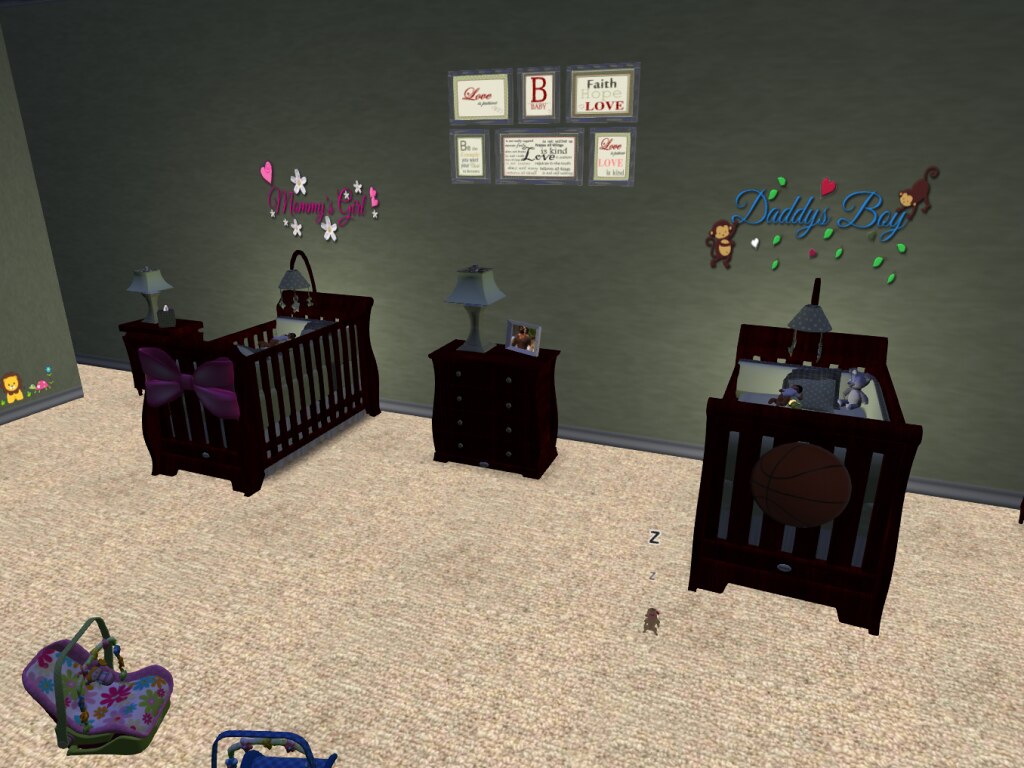In what appears to be a screenshot from a video game akin to The Sims or Second Life, we see a meticulously designed baby's room rendered with CGI graphics. The focal point of the scene includes two cribs positioned against a wall, flanking a nightstand placed in between. Above each crib, labeled signs denote "Mommy's Girl" for the crib on the left and "Daddy's Boy" for the one on the right. The "Mommy's Girl" sign is decorated with pink hearts, white flowers, and a hot pink bow adorning the front of the crib, while the "Daddy's Boy" sign features green leaves, playful monkeys, and a basketball at the front.

The nightstand that separates the two cribs holds a small lamp and an indistinct photograph. Further decorating the room, a grid of framed artwork hangs above the nightstand, displaying various motivational phrases like "Faith," "Hope," "Love," and "Be Safe." In the foreground, matching the thematic colors of the cribs, are two baby car seat carriers: one pink on the left and one blue on the right. This detailed and intricately arranged scene highlights a cozy and thoughtfully crafted virtual nursery.